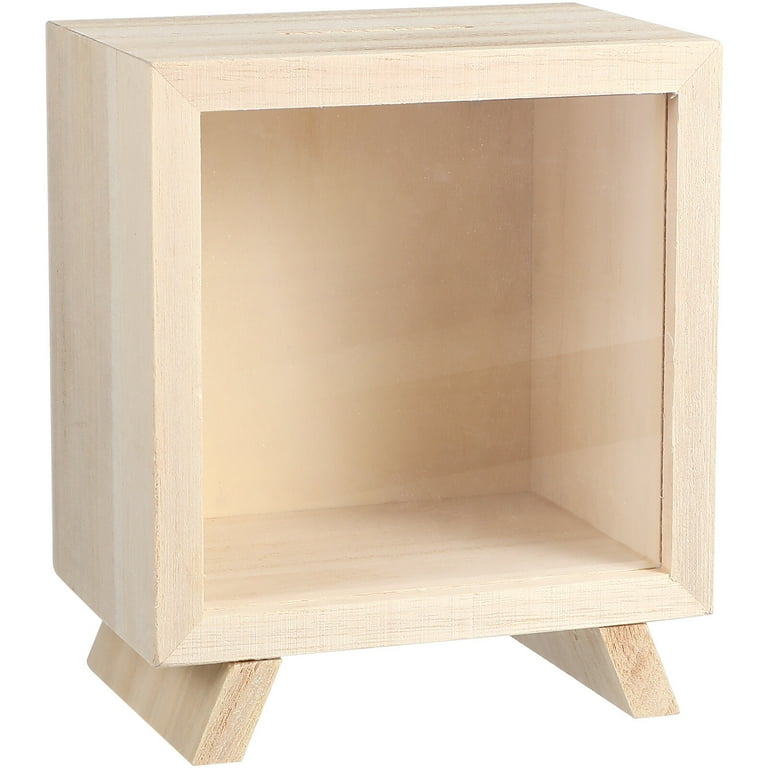The image is a photograph of a meticulously crafted, hollow, rectangular wooden box, aligned horizontally within an imaginary rectangle. The box, featuring a minimalist design that may hint at Japanese influences, is constructed from well-sanded, light tan wood with some darker tan accents. The smooth, unpainted surface suggests recent craftsmanship, possibly in the last decade. The box is open on the vertical plane from the viewer's perspective but closed at the back, with the orientation allowing someone to place items inside if turned on its side. It stands on two inward-turned wooden legs, made from the same light tan wood, providing stability. Enhancing its sleek design is a clear glass front panel that allows visibility into the interior, revealing subtle diagonal stripes, indicative of the wood grain or assembly technique. The overall impression is one of sturdiness and a nod to contemporary, minimalist design aesthetics, resembling an elegant, television-like cabinet.